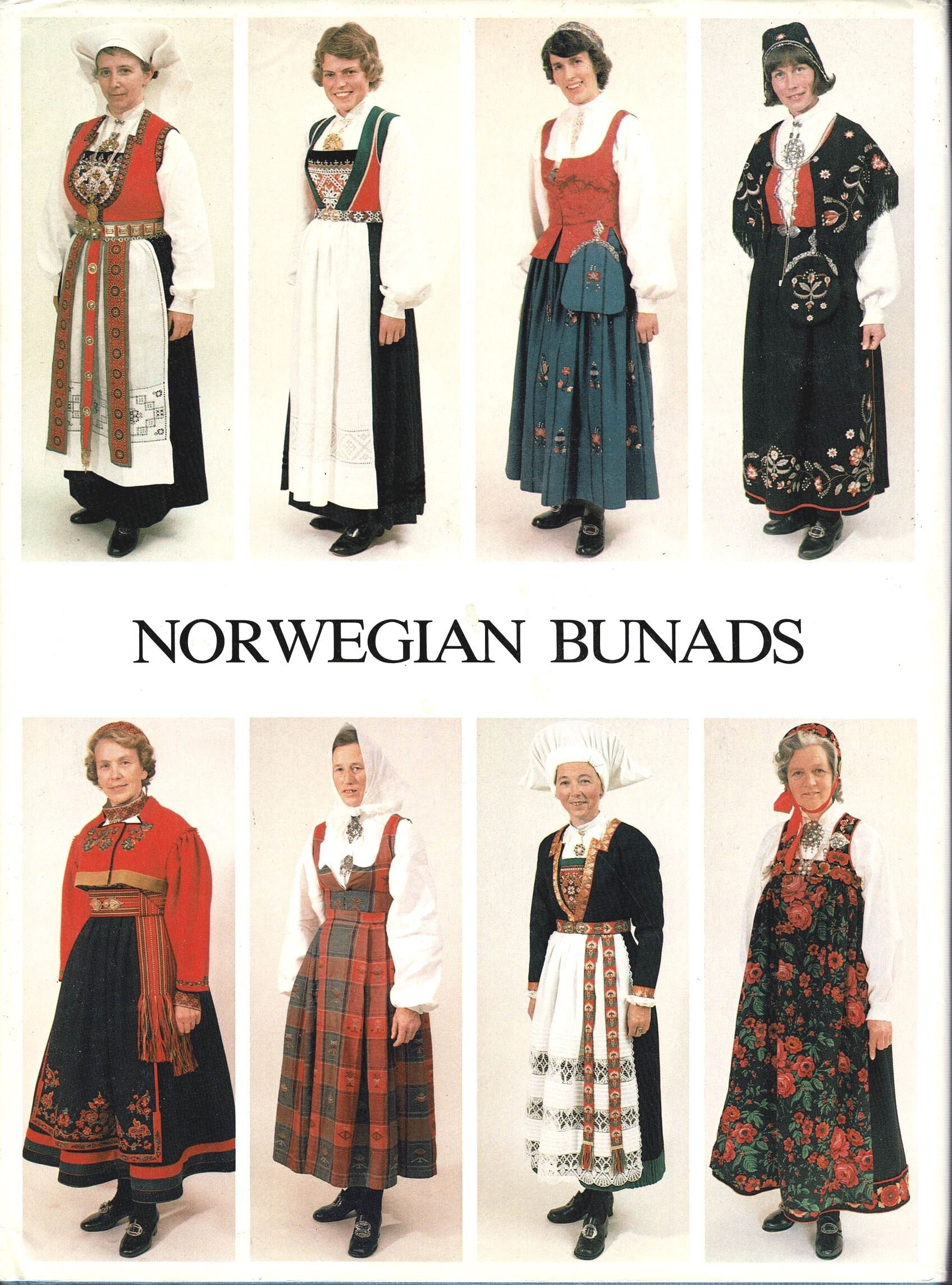The image appears to be a book cover or advertisement featuring the text "Norwegian Bunads" prominently in the center. Surrounding the text are eight equally spaced photographs of women dressed in traditional Norwegian ethnic clothing, arranged in two rows of four above and below the text. The women are adorned in vibrant, old-fashioned outfits, which include long-sleeved dresses that are modest and cover the entire body, often paired with aprons and corset tops or short jackets. The designs of the dresses vary from geometric patterns to floral and plaid, showing a combination of styles. Each woman is wearing black shoes, and some are carrying purses. Headwear ranges from bonnets and white hats to other hat styles. The women in the photos are of various ages, predominantly from their late 30s and onwards, and all are smiling warmly, adding a sense of happiness and amusement to the image. The overall layout with the text dividing the photographs, and the cheerful expressions on the women's faces, suggest a celebration of cultural heritage.